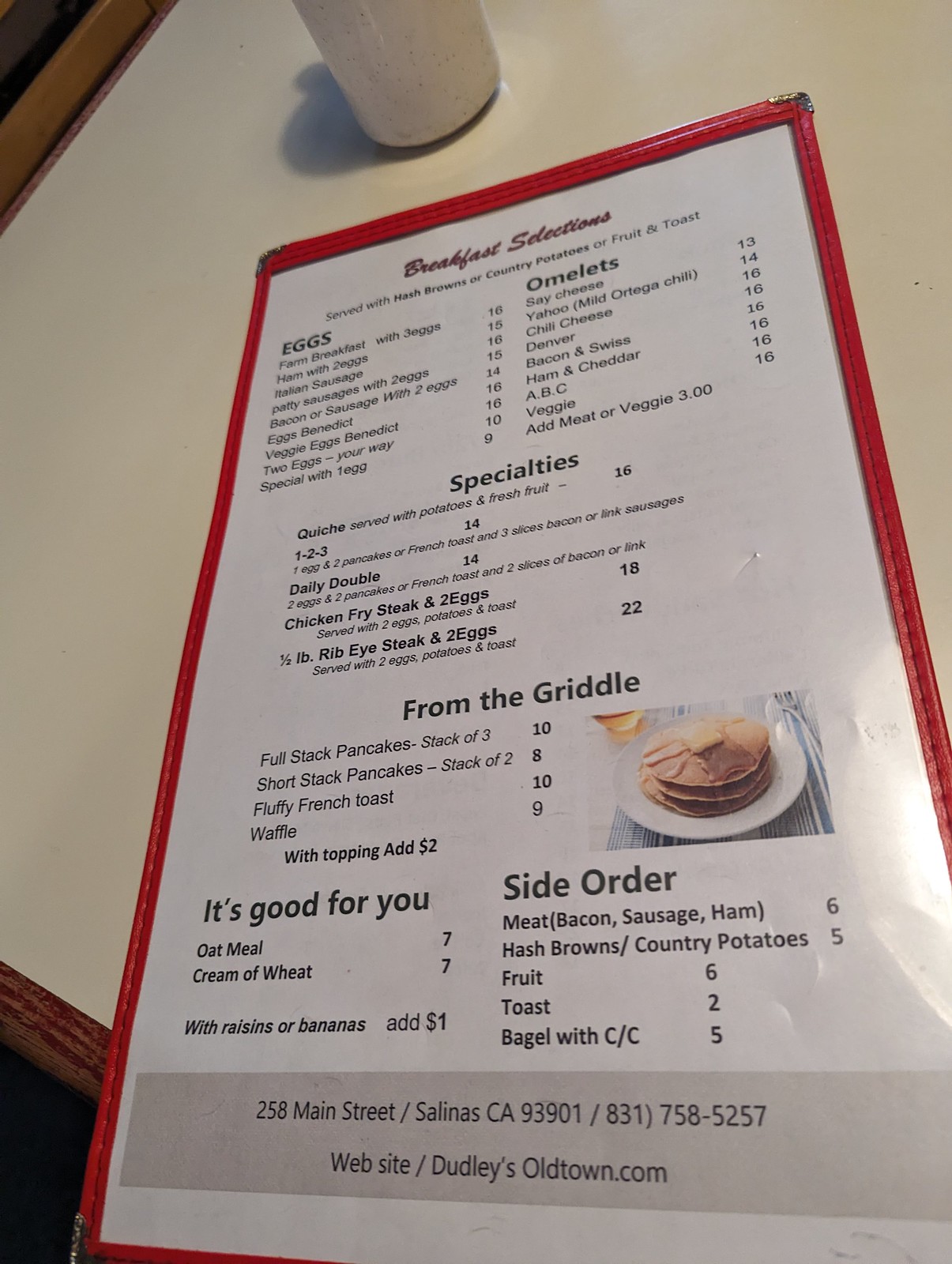A nostalgic scene captured inside a vintage 1980s-style diner. The setting features well-worn Formica or melamine tabletops, edged with orange-tinted, stained wood trim, characteristic of the bygone era. Centrally framed on the table is a menu encased in a clear plastic sleeve with a faux red leather binding and metal corners, evoking a sense of retro charm.

Beside the menu, a cup, possibly for coffee, casts a distinct shadow, suggesting an early morning visit. The menu itself offers a hearty selection of breakfast items, including hash browns, country potatoes, or fruit, served with toast. It features sections for eggs, omelets, specialties, and griddled delights like full stack and short stack pancakes, French toast, and waffles. A health-conscious section titled "It's Good for You" lists lighter options such as oatmeal and cream of wheat. The menu also includes a variety of side orders.

At the bottom of the menu is contact information for the establishment: 258 Main Street, Salinas, California 93901, with the phone number 831-758-5257 and the website deadliesoldtown.com. This image captures more than just a meal but a slice of timeless Americana.